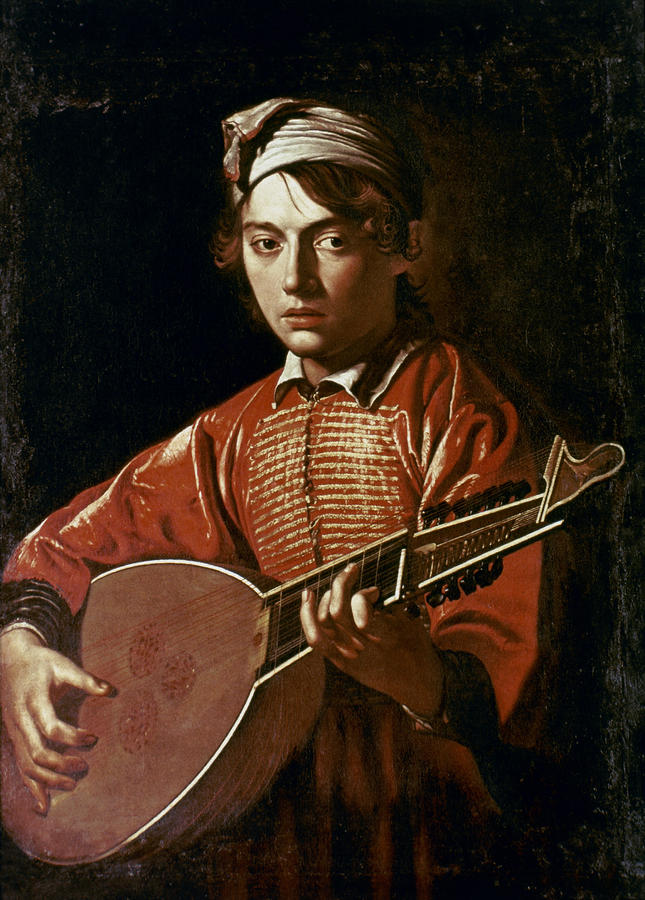The image depicts a detailed painting of a slightly melancholic young person facing the viewer, with their body turned slightly to the left, set against an abstract dark background that resembles a textured, grainy wall. They have reddish-brown hair partially covered by a white bandana or cap. The person is dressed in a striking red cloak or tunic, adorned with gold horizontal lines from the chest to the midsection, and black edging at the sleeves. They are intently playing an instrument that looks similar to a mandolin, featuring a distinct greenish-brown color with white borders and a large, rounded body. Their right hand is strumming while the left hand presses the chords on the instrument, which features multiple strings, possibly between 12 and 20. The overall scene is imbued with a somber, almost distraught feel, intensified by the deep, dark background.